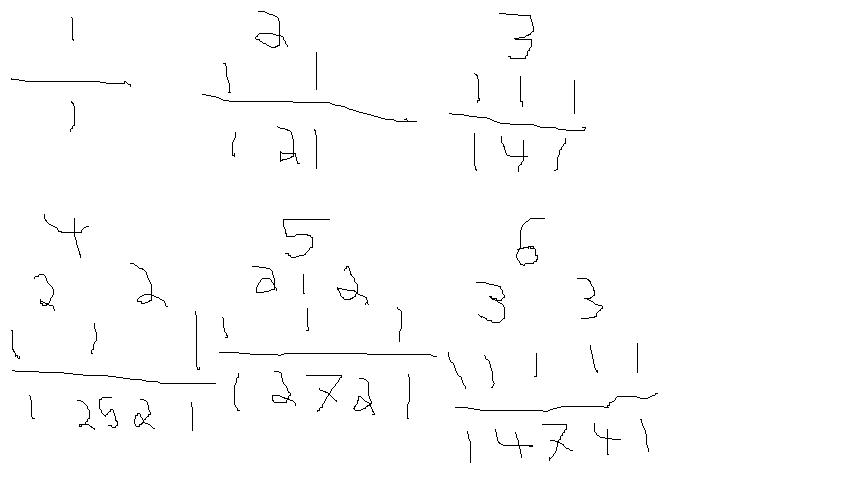The image displays a series of numeric expressions, neatly handwritten with either a pencil or pen on a white background. There are six distinct formulas arranged in an organized manner. 

- **Top Left**: The expression starts with the number '1', followed by a division line and another '1' below it.
- **Top Center**: The next formula features the number '2' over another '2', with vertical lines enclosing each '2'.
- **Top Right**: A '3' sits above a division line with a '4' beneath it, accompanied by three vertical bars above and two vertical bars flanking the '4' below.
- **Bottom Left**: This area contains the number '4', followed by the sequence '2, 2, 1, 1, 1'. A horizontal line underlines this set, and beneath the line, the sequence '1, 2, 5, 2, 1' is visible.
- **Bottom Center**: Here, we observe the number '5', followed by '2, 1, 2, 1, 1, 1' in sequence, with a horizontal line underneath. The formula continues with '1, 2, 7, 2, 1' after the line.
- **Bottom Right**: The final formula starts with '6' and is followed by '3, 3, 1, 1, 1, 1, 1', ending with a horizontal line, and below the line numbers '1, 4, 7, 4, 1' are displayed.

This carefully composed set of formulas showcases a blend of division and pattern within the handwritten notation.